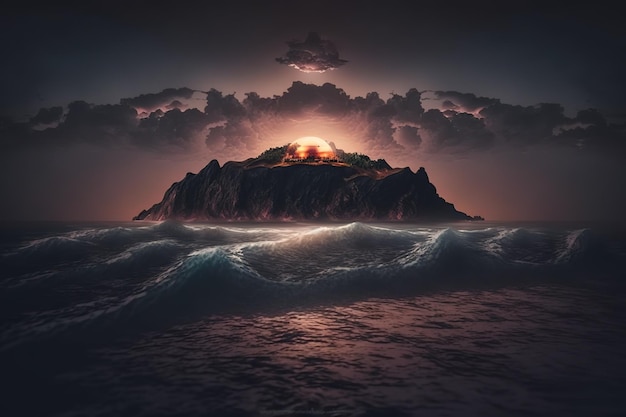The image is a detailed piece of digital art that captures a surreal and captivating scene in a twilight setting. The bottom half of the image shows ocean waves receding from a beach toward an island at the center. Dominating the island is a glowing, yellow dome—though it could also be an energy field pulsating outward—that illuminates the surrounding area and creates a bright aura in the sky above. This light bathes the clouds directly overhead in a radiant hue, almost as if a beam of light is shooting through them. The sky is a contrasting mix of dark, thick clouds and a pinkish glow, giving the scene an ominous yet enchanting atmosphere. The symmetry of the clouds across a vertical axis adds to the visual balance. The overall color scheme is dark and brooding, with touches of gray and pink light, skirting between the realms of awe and foreboding.